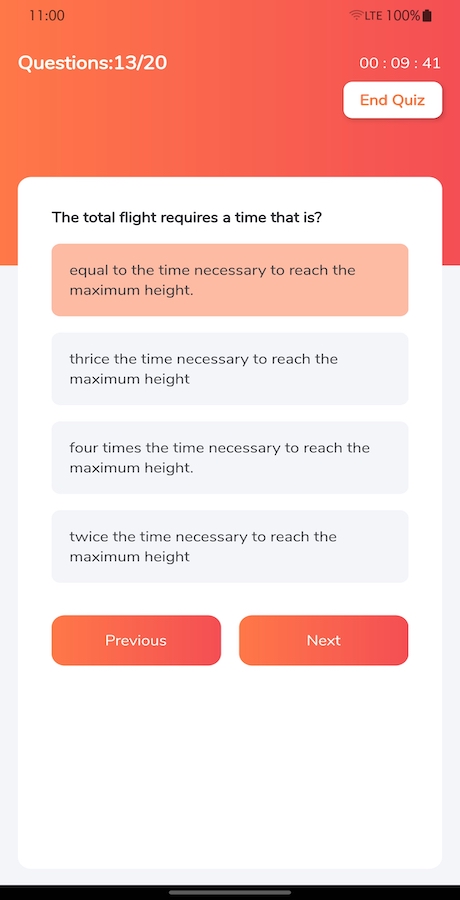This image is a detailed screenshot from a mobile quizzing app. In the upper right corner, the phone's battery is fully charged at 100%. The quiz interface prominently features a rectangular box at the top in an orangey-red color, containing the text "Questions: 13/20" in white. Below it, a timer displays "00:09.41". Adjacent to the timer, a white bubble with pinkish lettering reads "End Quiz". 

Beneath this, there is a vertical white box extending into the orangey-red horizontal box, which presents the current quiz question. The question, written in bold text, is: "The total flight requires a time that is ?". Below this, there are four multiple-choice answers: 
1. Equal to the time necessary to reach the maximum height.
2. Thrice the time necessary to reach the maximum height.
3. Four times the time necessary to reach the maximum height.
4. Twice the time necessary to reach the maximum height.

The first option is highlighted in light pink, indicating it has been selected by the user. At the bottom of the question box, there are two buttons in orangey-red with white text: "Previous" on the left and "Next" on the right.